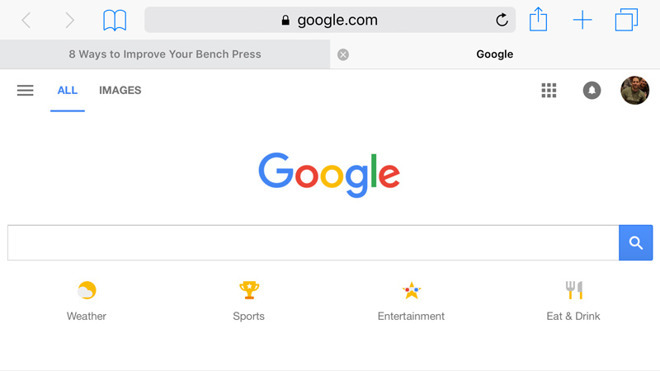This screenshot features an iPhone displaying the Safari web browser with two open tabs. The primary tab, currently in focus, displays the Google homepage. The iPhone is positioned horizontally, providing a widescreen view of the content. 

The Google homepage showcases a clean, white background adorned with the Google logo in the center, featuring its iconic blue, red, yellow, and green colors. Above the logo is a gray UI header bar which includes a hamburger menu at the upper left corner. Just beneath the Google logo is a search bar that spans the entire width of the screen, complete with a blue search button on the right, highlighted by a white magnifying glass icon.

Directly underneath the search bar, there are four evenly spaced elements labeled "Weather," "Sports," "Entertainment," and "Eat & Drink." Each section features a distinctive icon: a yellow sun behind white clouds for Weather, a golden trophy for Sports, a white star with 3D glasses for Entertainment (with one red and one blue lens), and a gray fork and knife with orange handles for Eat & Drink.

The secondary tab, titled "Eight Ways to Improve Your Bench Press," is also visible but not highlighted.

Every detail contributes to a user-friendly and visually organized layout, typical of Google's clean design and intuitive interface.